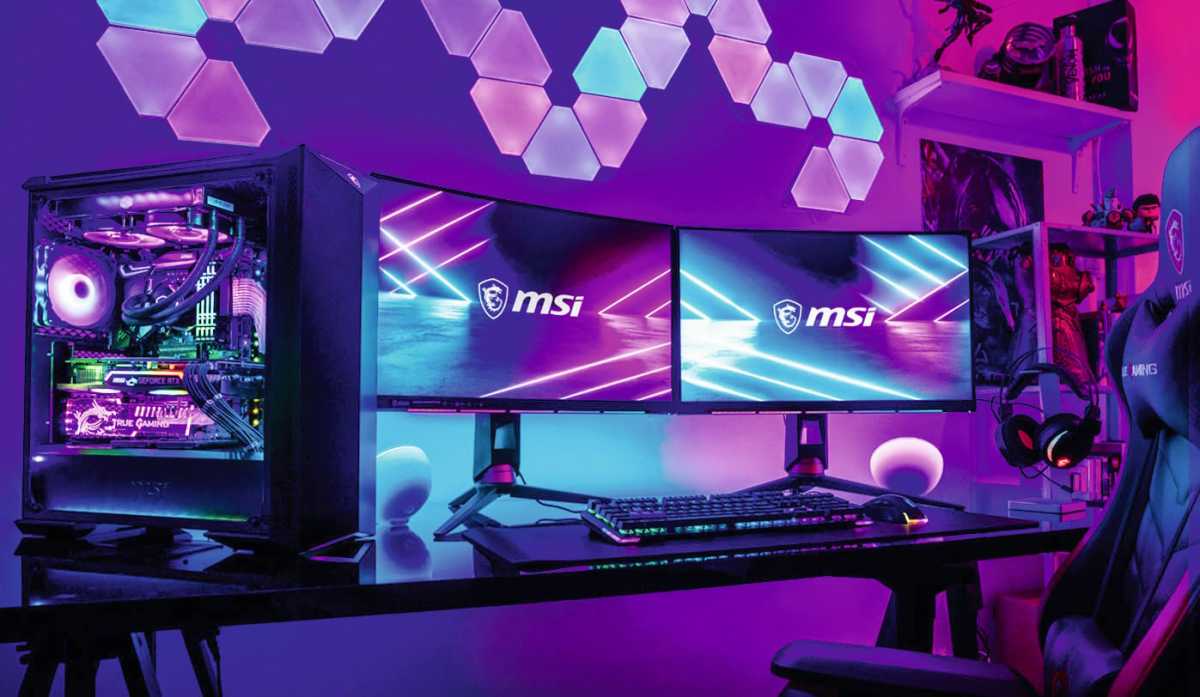This image showcases a highly detailed and aesthetically striking gaming setup. On the left side, a black open computer case reveals its glowing internal components, illuminated primarily in shades of purple and blue, with accents of green. Visible inside are large fans, including one on the left and others on the top connected to a radiator for liquid cooling the processor, with noticeable lines extending from the radiator to the processor. The power supply at the bottom connects to a vividly lit, rainbow-colored video card. Centered in the setup are two MSI monitors of the same size, slightly angled outward, with the MSI logo prominently displayed. The monitors rest on a dark desk that houses a black keyboard emitting rainbow lights from its base, a gaming mouse, and two circular Bluetooth speakers positioned beneath the screens.

A black gaming chair with red details sits partly rolled away from the desk. A headset stand with partly lit headphones accompanies the setup. Overhead, the wall features modular LED lights forming a sideways S-like pattern, displaying hues of pink, purple, and blue, contributing to the room's futuristic and synthwave ambiance.

To the right of the desk are shelves containing various objects, including what might be figures and a bottle on the top shelf. These shelves share space with a square shelving unit adorned with additional figures and unidentifiable items, all set against a poster on the wall. Overall, the room exudes a sense of advanced technology and vibrant visual appeal, heavily influenced by the blend of purple, blue, and pink lighting themes.